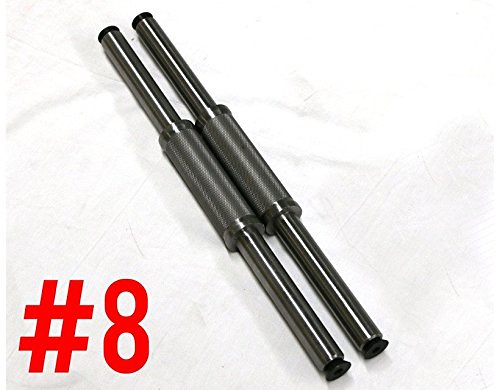The photograph showcases two cylindrical, metallic objects lying diagonally on a white linen fabric. These objects each feature a central thicker cylinder from which thinner rods extend, resembling a potential exercise tool or mechanical component. Both rods have small black plastic loops or rubber pieces at their ends. The reflective surfaces of these objects suggest they could be constructed from iron or similarly shiny material. They are positioned with the bottom right towards the viewer while the top left angles away, hinting at a perspective shift. Intriguingly, the bottom left corner prominently displays a large red hashtag "8", adding a graphic element to the otherwise mechanical scene. The overall setting implies a clean, possibly soft background, made ambiguous by its shadows and texture.